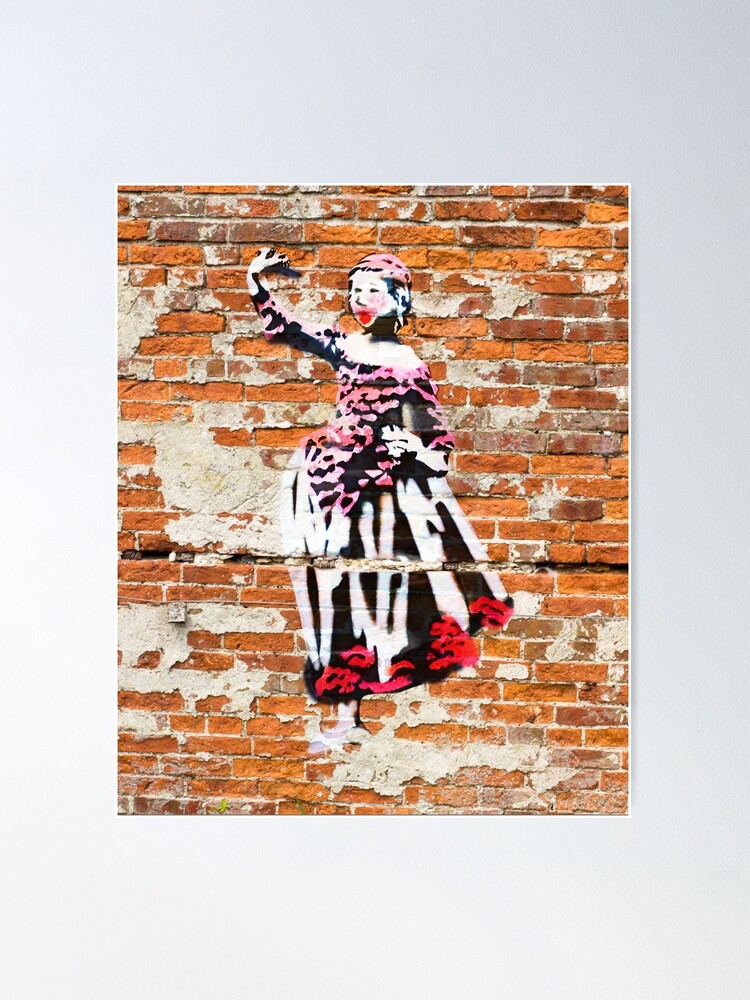This captivating artwork portrays an urban brick wall adorned with remnants of peeling plaster, revealing hints of the wall's past. Central to the piece is a striking black and white graffiti image of a young girl in a dress. She gazes thoughtfully to the left, her hand raised in an expressive gesture. Despite the grayscale palette, the artist has added striking details in color: a touch of pink graces the upper part of her dress, while sporadic red blobs accentuate the lower portion. The graffiti's meticulous execution gives it a photographic quality, almost as if it's a printed poster seamlessly integrated into the urban landscape, blurring the lines between street art and traditional art forms.